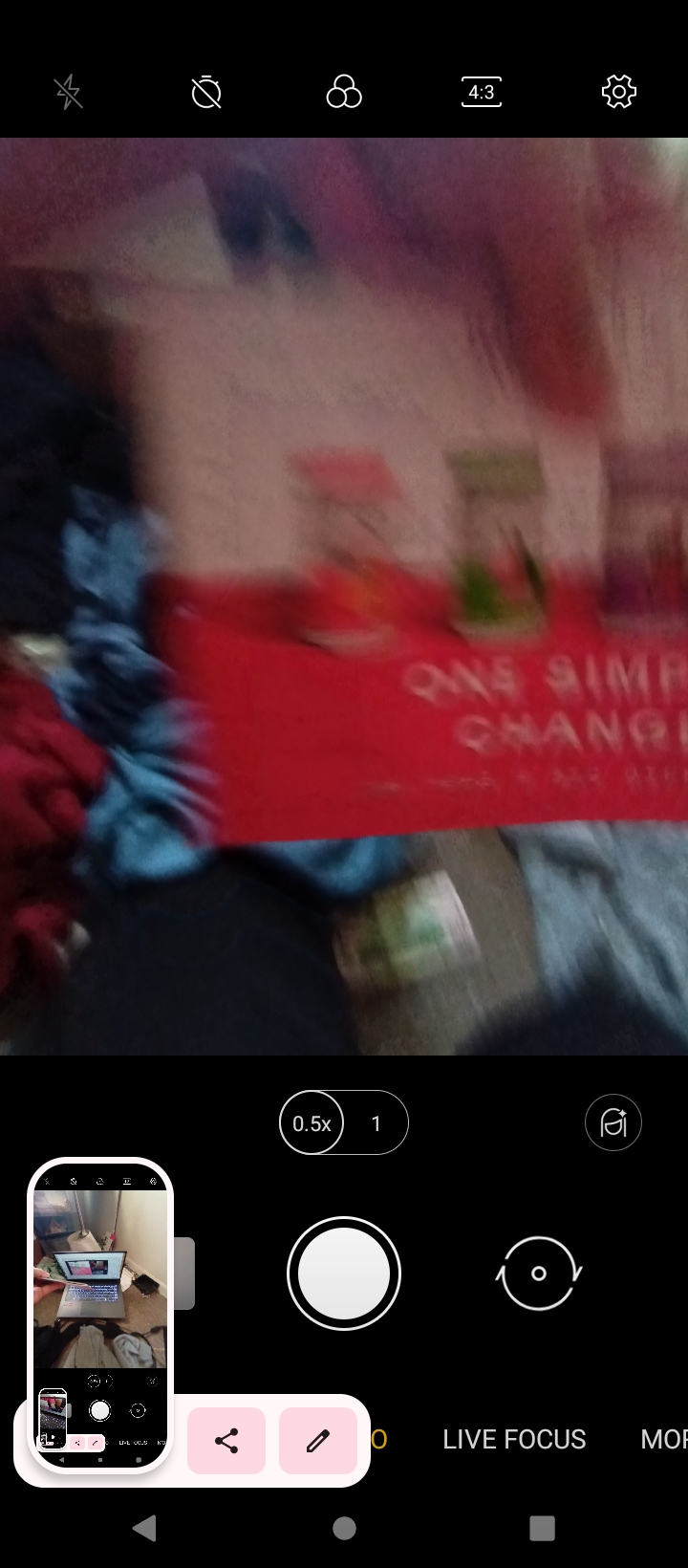This image is a blurry screenshot, possibly from an Android cell phone, capturing the camera app interface. The screen is framed by typical cell phone icons, with the standard white button for taking a picture centered at the bottom. The lower third features black borders with the "Live Focus" label in white capital letters on the right. An oval icon with "0.5X" and "1" options suggests the camera’s zoom capabilities. In the lower left corner, there's a smaller, inset image revealing a cell phone camera screen aimed at a laptop in front of a living room setting.

The main image depicts a person holding a red and white package, although the details are obscured due to the blurriness. Visible text on the package reads "one simple change," though the last few letters are cut off. Surrounding the person, the scene includes bottles or jars set on a mantel, which is partially draped with a red cloth and backed by white-painted brickwork. There are some crumpled clothes visible on the floor, adding to the cluttered appearance of the room. Despite the blurry focus on the main subject, the camera app's icons and interface remain sharp and clear.